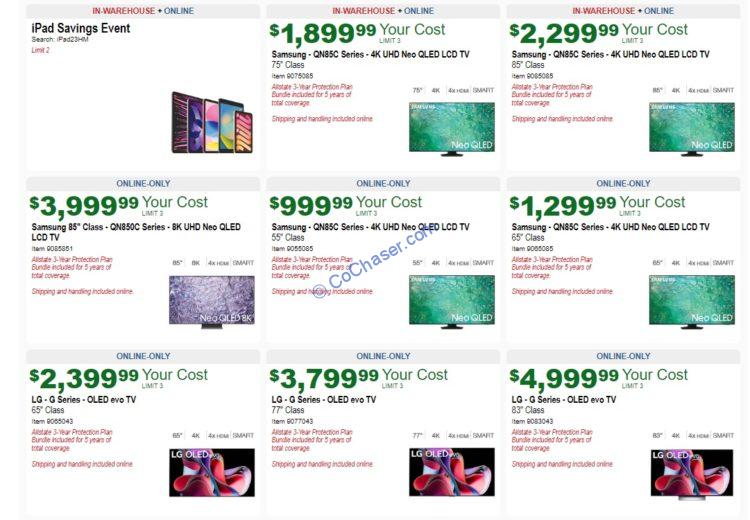The image is a promotional collage of various tech items organized in a grid with three rows and three columns. Each item is displayed in a rectangular section that features a white background with a gray border at the top. The top border of each rectangle is labeled with "In-House" in red and "Online" in blue for the first three items, reading left to right.

In the first row, the upper left rectangle includes text in black stating "iPad Savings Event Search," highlighting an iPad model identified as "Pad 23, HM" with a purchase limit of 2 units denoted in red. A picture of the iPad is also present within this section.

The next rectangle in the first row features a Samsung QNC B85C Series 4K UHD Neo QLED LCD TV, 75-inch, priced at $1,899.99, with the price displayed in green text. 

The last rectangle in the first row repeats the Samsung QNC B85C Series details, this time featuring an 85-inch TV priced at $2,299.99, also with a limit of 2 units indicated in black text.

In the second row, the first rectangle advertises another Samsung 85-inch TV. The second rectangle showcases a Samsung 55-inch TV, and the third displays a 65-inch Samsung TV. 

In the final row, the first rectangle highlights a 65-inch LG Series TV. The second rectangle lists a 77-inch LG Series TV, and the last rectangle describes an 83-inch LG Series TV.